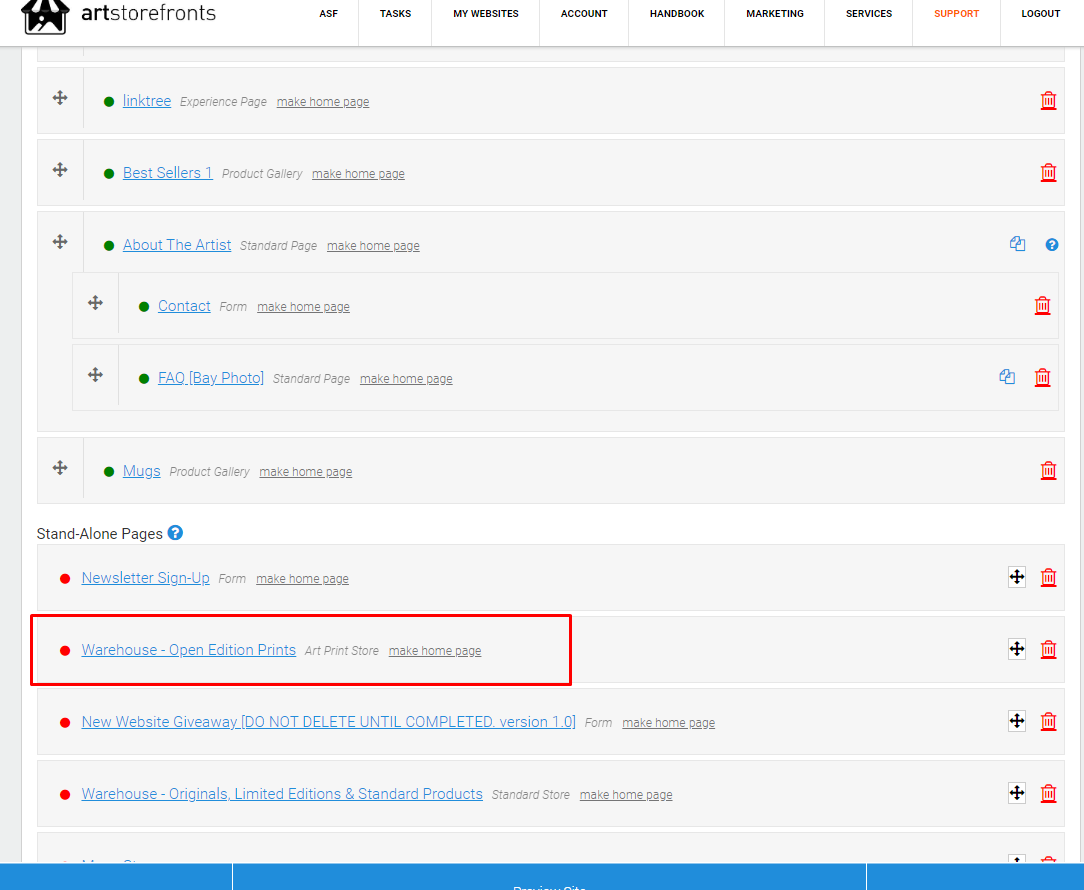The image captures a minimalist yet technical screenshot from a platform named "ArtStorefronts." The user interface depicts a tent-like setup akin to a carnival booth, emphasizing the platform's simplicity and user-friendliness. The top navigation bar includes tabs such as ASF Tasks, My Websites, Account, Handbook, Marketing, Services, Support, and Log Out. 

The current section is 'Support,' showcasing various interactive elements and links. Noteworthy links include "Link Tree," alongside clickable options like "Make Home Page." This feature is available for all items listed. Other links visible are "Bestsellers," "About the Artist," "Contact," "FAQ," "Mugs," "Standalone Pages," "Newsletter Signup," "Warehouse," and "New Website Giveaway." 

A distinct box highlights the "Warehouse" and "Open Edition Prints" links, suggesting a focus on organizing or prioritizing these sections. The overall scene hints at a merchant configuring their online storefront, fine-tuning the presentation and functionality to enhance their website’s usability and aesthetics.